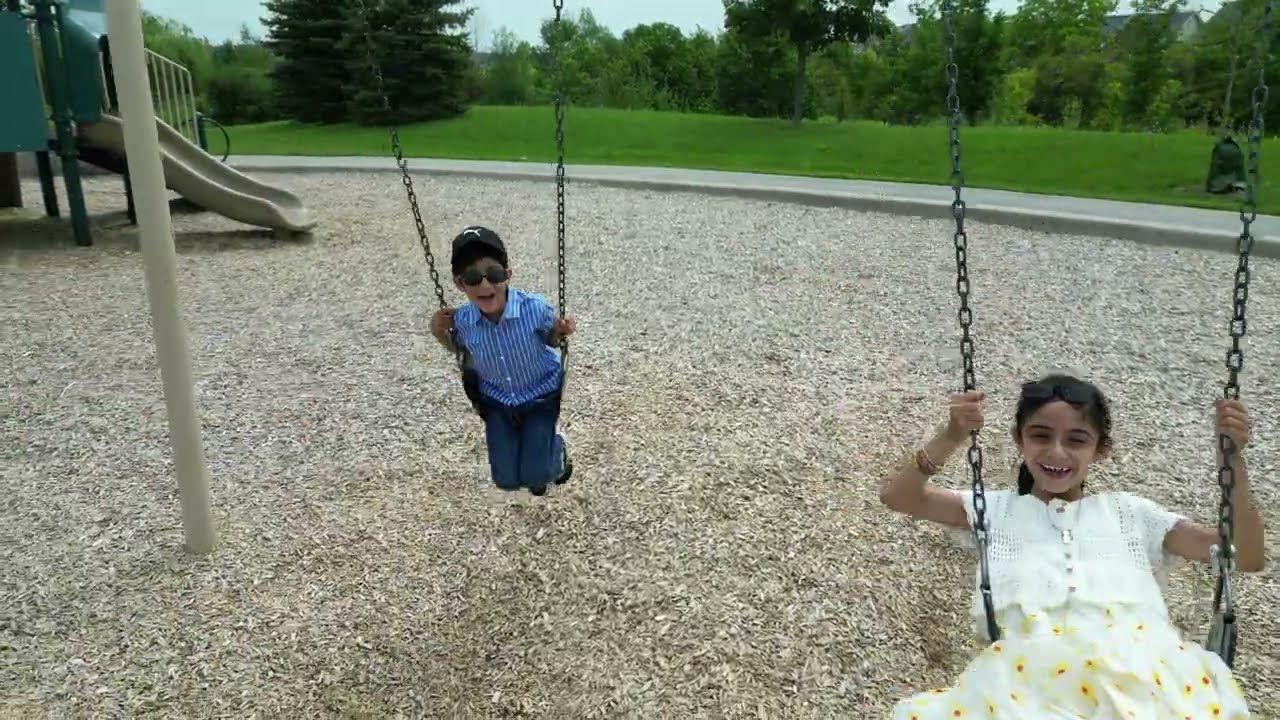In this vibrant image taken at a park, two children are joyfully swinging on a tan-colored swing set surrounded by light-colored wood mulch. The scene captures a sunny day with lush green grass and large pine trees creating a natural backdrop. On the right side, a young girl with medium skin tone and brown hair tied back into a ponytail is wearing a charming white dress adorned with yellow flowers. She is holding onto the swing chains, leaning forward with a big, open smile, as if laughing. On the left, a young boy dressed in a white and blue striped button-up shirt, blue jeans, a black ball cap, and sunglasses swings in the opposite direction, also with an open-mouthed smile indicative of laughter. Behind the children, a slide is visible in the upper part of the photograph, further emphasizing the playful atmosphere of the park setting.